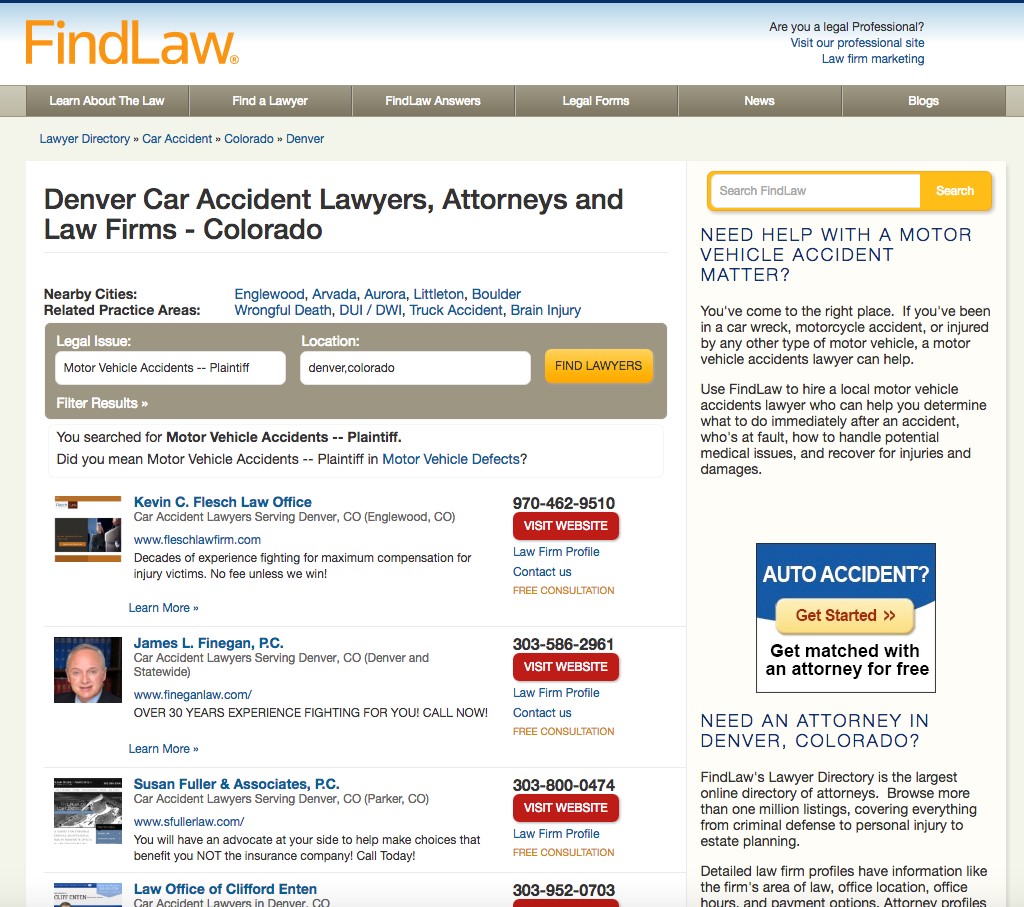The image showcases a legal referral website branded as "FindLaw," prominently featuring its logo in orange against a light blue header in the top-left corner. Below the header, a navigation menu offers several options: "Learn About the Law," "Find a Lawyer," "FindLaw Answers," "Legal Forms," "News," and "Blogs," arranged from left to right. Centered on the page is the title "Denver Car Accident Lawyers, Attorneys, and Law Firms Colorado," indicating a localized legal service for Colorado.

To the right of this title, a search bar labeled "Search FindLaw" allows users to explore the site. Below this, a comprehensive search box titled "Legal Issue" enables visitors to enter various legal issues and locations, with a "Find Lawyers" button for execution. Additionally, a "Filter Results" button is located at the bottom of this box for refined searches.

The lower section of the page displays profiles of multiple attorneys, including their websites and phone numbers, facilitating direct contact. This detailed layout aims to assist users in navigating and selecting legal services specifically tailored to their needs in Colorado.